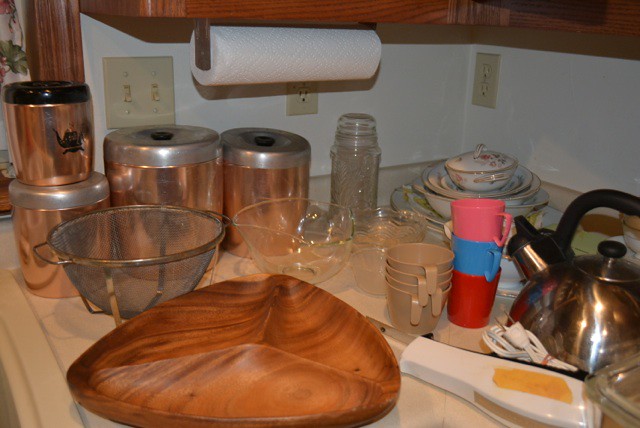The image is a richly detailed color snapshot of a bustling kitchen countertop corner. The countertop, appearing either white or tan, is cluttered with various objects, giving it a lived-in, homey feel. Framing the photo are glimpses of wood from wall-mounted cabinets on both sides. The left cabinet, positioned centrally at the top of the image, features an under-cabinet mounted paper towel holder with a roll in place. Behind this, an ivory or almond-colored electrical receptacle is visible. There's a matching receptacle on the adjacent wall, accompanied by double light switches of the same color on the left.

The wall space between the cabinets and the countertop is painted white, providing a clean backdrop for the assortment of items below. In the foreground stands a unique triangular-shaped, divided wooden serving tray, possibly made from teak wood popular in the Philippines, known as monkey puzzle wood. To its right, a white plastic object with a plug -- potentially an electric knife -- is partially visible. Adjacent to this is a sleek, stainless steel (or chrome) tea kettle with a black handle and black knob.

A stack of plastic cups with handles is placed next to the kettle, arranged in a red, blue, and pink sequence from bottom to top. To the right of these cups is another stack of tan plastic cups, featuring partial handles that extend out and downward. Nestled in the corner is a stack of china, adorned with pink or red flowers and gold trim. This collection includes a covered bowl or terrine with strap-like handles, nested serving bowls, and a shallow bowl, all atop a platter.

Further in the background, a glass canister with an airtight lid sits to the left of the china stack. Beside it is a vintage aluminum canister set, mid-century styled with a copper-colored bottom and plain aluminum lids featuring black knobs. Notably, an odd smaller canister with a black lid and a black design, potentially a tea kettle, sits atop the leftmost canister.

Rounding out this eclectic mix are a mesh strainer or colander and some glass bowls, adding to the array of kitchen essentials. This snapshot captures the charm and character of a well-used and loved kitchen space.